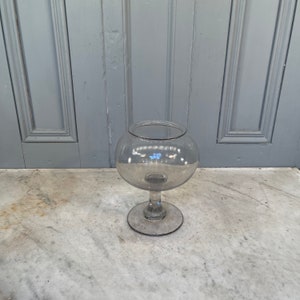This image features a light green, transparent margarita glass with a wide bulbous bowl and a circular opening at the top, situated in the center of the photograph. The glass has a distinctive wide base and a slender stem connecting it to the cup portion. The setting appears to be in an indoor space, placed atop a marble countertop characterized by a darker color palette of gray interspersed with light brown and dark gray swirls. In the background, grayish-blue cabinets add to the scene's aesthetic. Reflections within the glass hint at multiple light sources, potentially resembling ring lights. The marble countertop's intricate pattern is prominently visible, and the blue-grayish hues of the surroundings further complement the ambiance.